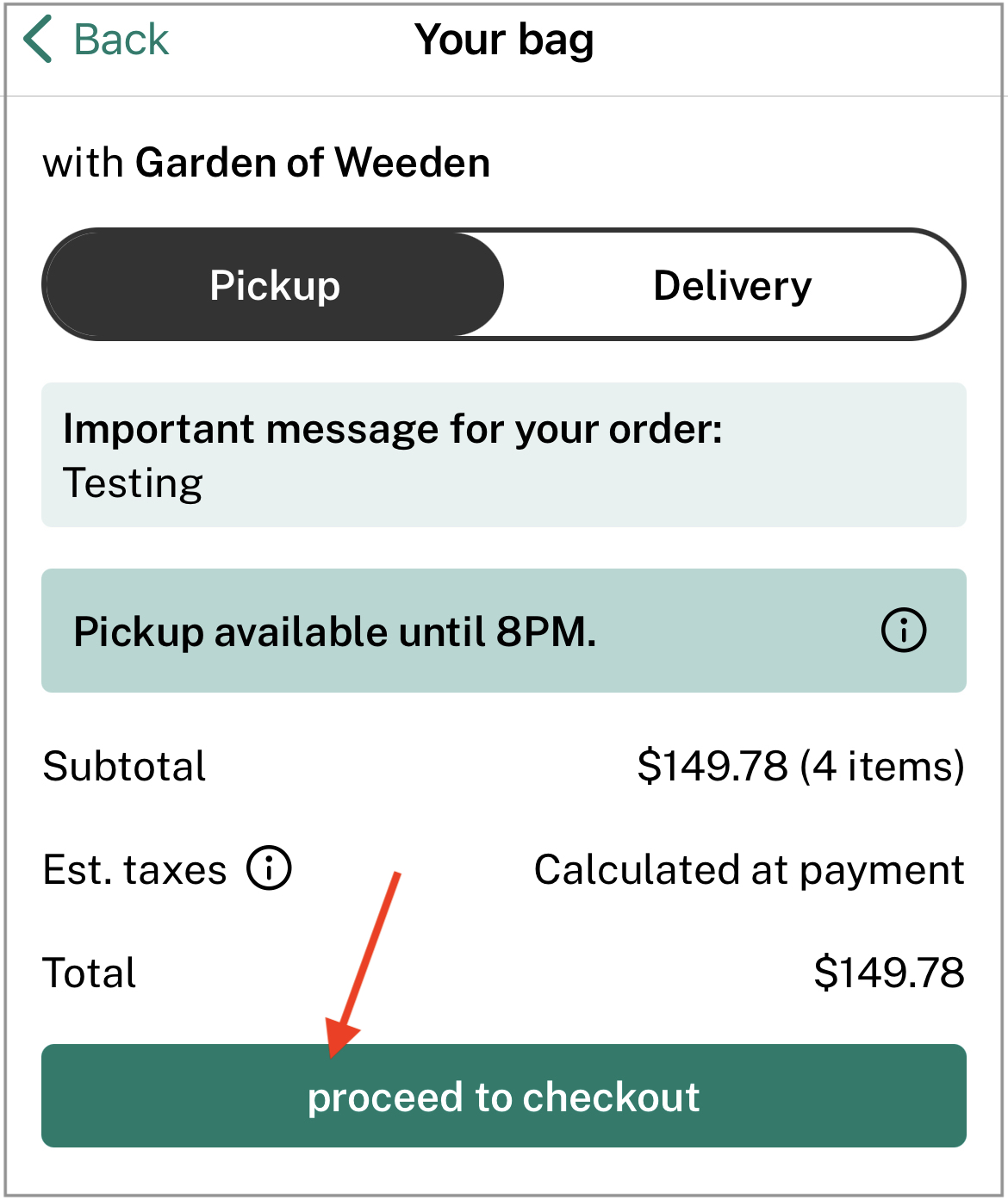Screenshot of a cell phone or computer window displaying shopping cart details. In the top-left corner, there's a green arrow pointing left, accompanied by the word "Back." Centrally located on the screen is the label "Your Bag," with a subtitle "with Garden of Weden" just below it. Further down are two buttons, "Pickup" and "Delivery," with "Pickup" highlighted. 

An important message for the order is displayed in a green rectangle, stating "Important message for your order testing." Beneath it, another green rectangle indicates "Pickup available until 8pm," accompanied by an informational button to its right. 

The subtotal for the items is $149.78, highlighted in black text below the green rectangle. The estimated tax will be calculated at payment. 

The total amount is $149.78, clearly displayed. A red arrow points downwards to the bottom of the screen, directing attention to a green rectangle button labeled "Proceed to Checkout."